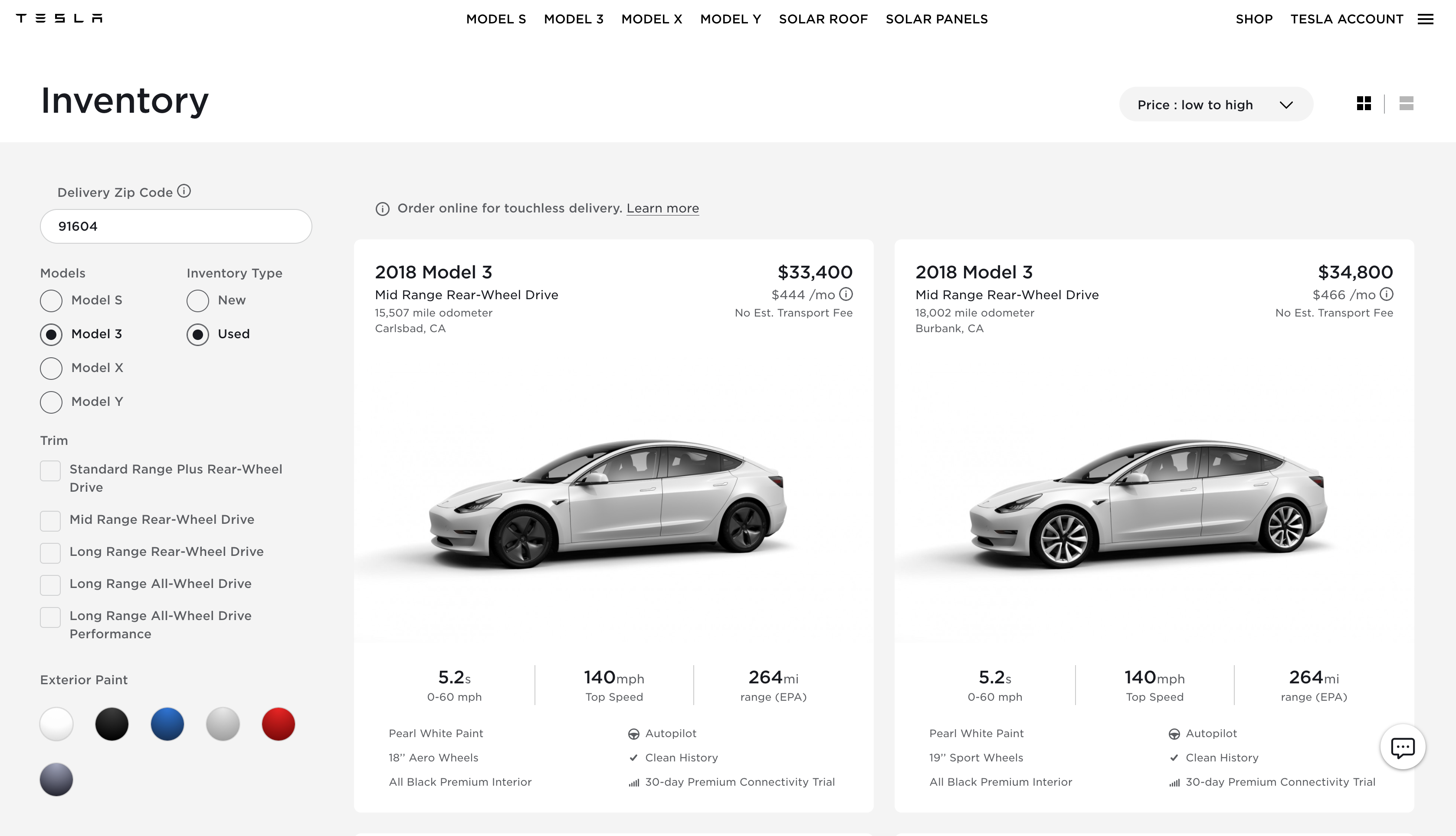In the top left corner of the image, the word "Tesla" is prominently displayed. To the right, the options for "Model S," "Model 3," "Model X," "Model Y," "Solar Roof," and "Solar Panels" are listed sequentially. Further to the right are options to "Shop" and access your "Tesla Account." Just below these headings on the left, the word "Inventory" appears next to a circle enclosing the text "Delivery Zip Code 91604." Beside this, there are black circles indicating selections for "Model 3" and "Inventory Type Used."

On the right side of the image, inside a white square, a 2018 Tesla Model 3 is featured, listed at $33,400. This vehicle boasts a top speed of 140 miles per hour and a range of 264 miles. Another similar vehicle is displayed to the right, appearing slightly lighter in color, priced at $34,800. Both vehicles share the same performance specifications: a 264-mile range and a 140 miles per hour top speed.

To the far left, there's an "Exterior Paint" option with various color circles available, including white, black, blue, gray, silver, and dark gray.